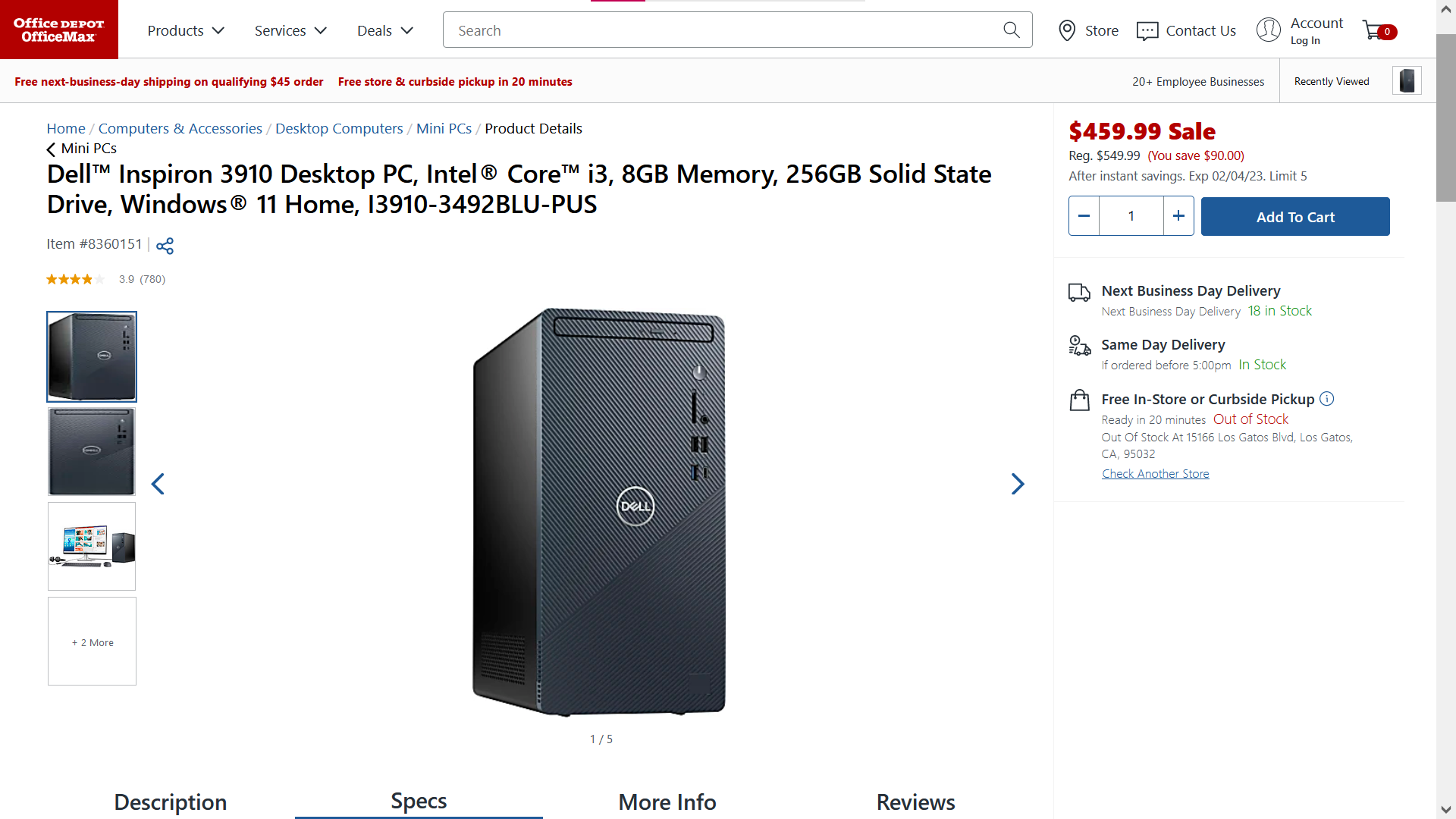Here is a cleaned-up and detailed caption for the image:

---

For sale is a Dell Inspiron 3910 Desktop PC, prominently listed on the Office Depot Office Max website. In the top left corner, a red box features the store's name, while the navigation bar includes options for Products, Services, Deals, a search bar, store locator, contact us, account login, and a shopping cart icon. Below, highlighted offers include free next-day shipping on qualifying $45 orders and free store and curbside pickup within 20 minutes. 

The product is categorized under Home, Computers and Accessories, Desktop Computers, Mini PCs. The item on display is a Dell Inspiron 3910, Desktop PC equipped with an Intel Core i3 processor, 8GB of memory, and a 256GB solid-state drive, running Windows 11 Home. The model number is i3910-3492BLU-PUS. 

A clear image of the product is accompanied by several thumbnail images on the left side of the page. On the right, the sale price of $459.99 is prominently displayed in red, reduced from the regular price of $549.99, giving buyers a $90 savings after instant savings. The offer is valid until 02-04-23, with a purchase limit of 5 units. Below, users see an "Add to Cart" button next to a quantity selector set at 1.